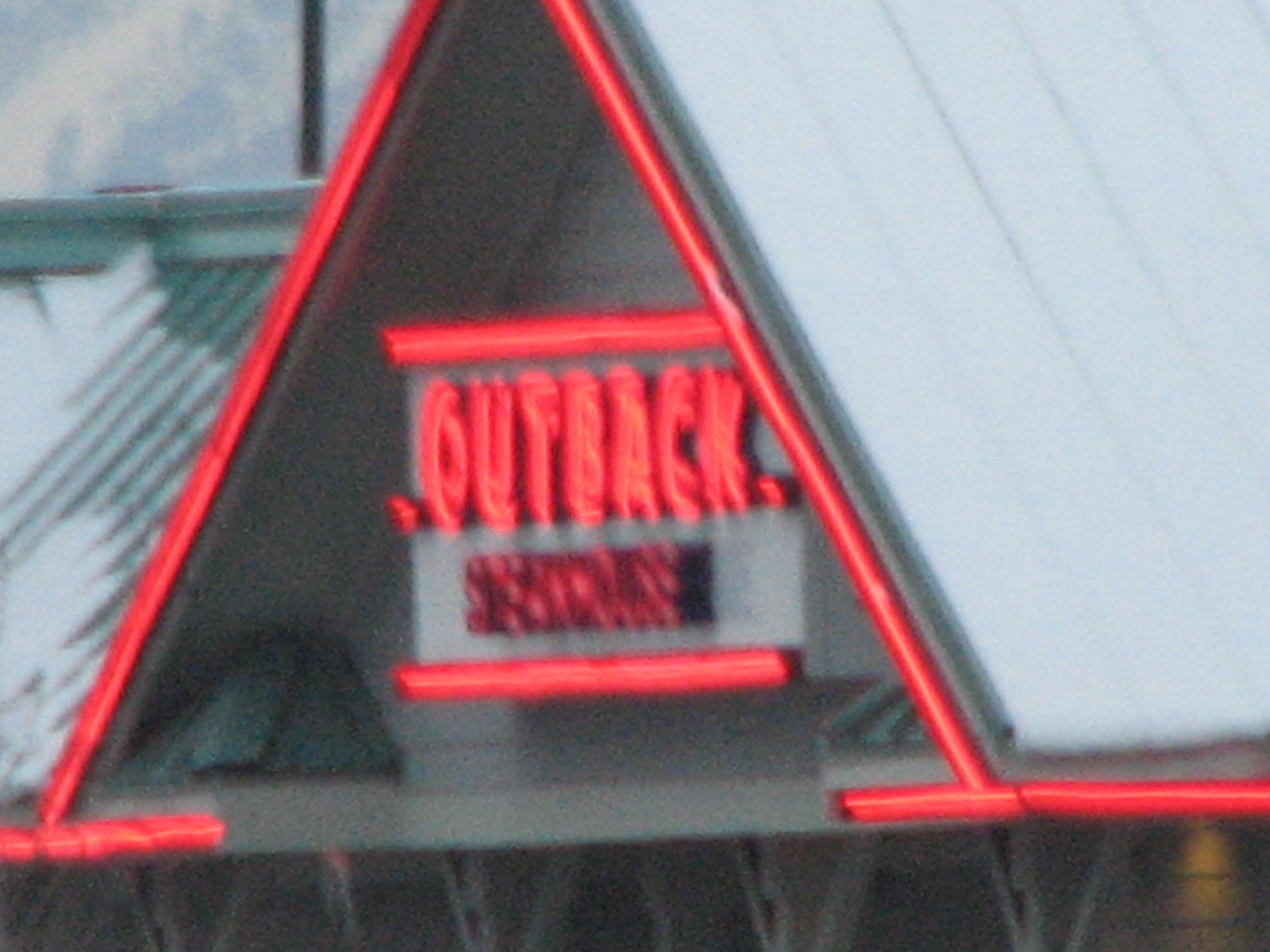This is a close-up, blurry, and grainy photo of the sign at the entrance of an Outback Steakhouse. The building features a triangular roof painted in a very pale robin's egg blue or gray color, topped and outlined with bright red neon lights that form a triangular shape around the roof but do not reach the peak. The red neon lights are activated, creating an illuminated effect. The primary focus of the image is the Outback Steakhouse sign, which is visibly three-dimensional with "Outback" written in large capital letters above “Steakhouse,” which is considerably smaller. Both words are in bright neon red. Above “Outback” is a thick red neon line, mirrored by a thinner red line below “Steakhouse.” Some structural supports beneath the roof are faintly visible, and there’s an overcast sky in the background with a hint of snow on the left side of the roof. The context of the lower part of the building and the entrance is not visible in this photo.